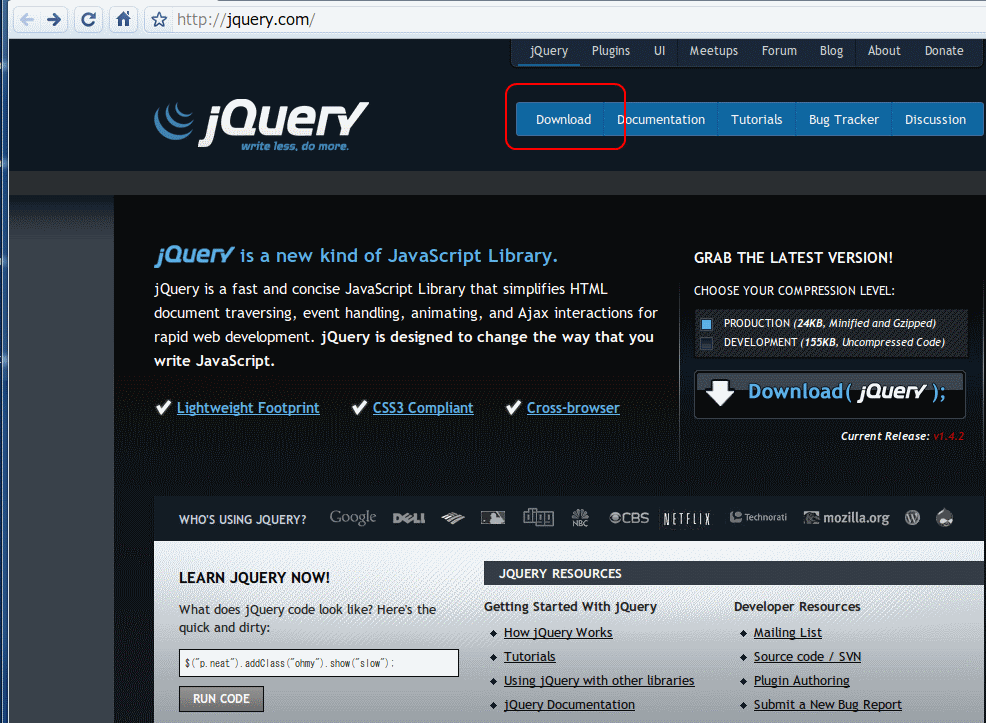This screenshot captures the homepage of the jQuery website, accessed through the URL http://jquery.com/. The interface is organized with a structured layout beginning with the browser's address bar at the top. Directly below, a navigation menu is presented, and underneath that, another menu is displayed on a blue bar with white text. This secondary menu includes options labeled: Download, Documentation, Tutorials, Bug Tracker, and Discussion. Notably, the Download option is emphasized with a red oval drawn around it.

The main content area of the page features a striking black background contrasted with blue and white text. In the upper left-hand corner, the jQuery logo is prominently displayed along with the slogan, "Write Less, Do More."

The central portion of the page introduces jQuery with the phrase, "jQuery is a new kind of JavaScript library," followed by prompts for the user to grab the latest version and choose their compression level. A prominent Download button is also featured here.

Towards the bottom of the page, a light gray rectangular menu offers additional resources under the heading 'jQuery Resources,' including sections for 'Getting Started with jQuery' and 'Developer Resources.' In the lower left-hand corner, there is a call to action with the phrase "Learn jQuery Now," accompanied by a “Run Code” button.